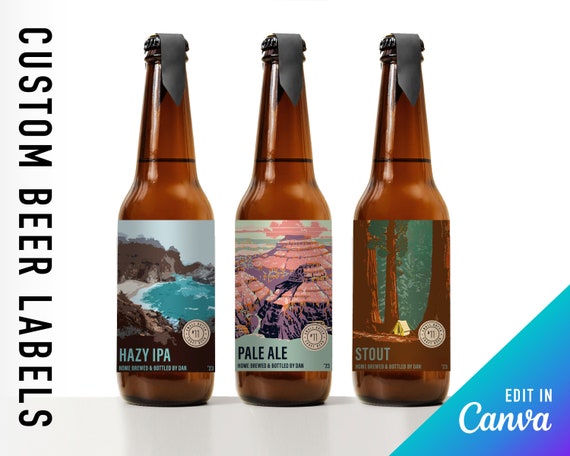This is a vibrant color image that appears to be an advertisement for a beer label manufacturer. At its center are three brown glass beer bottles, each filled with clear liquid and topped with black caps sealed by an additional dark gray element wrapped over the top. The backdrop is a clean, white surface, and the bottles rest on a gray foreground. 

To the left of the bottles, vertical black text reads "Custom Beer Labels," while on the bottom right, a blue triangle banner features white text that says "Edit in Canva." Each bottle prominently displays a unique custom label. The leftmost bottle showcases a beach scene with the text "Hazy IPA" in blue at the top. The middle bottle exhibits a southwestern Grand Canyon-like landscape with "Pale Ale" inscribed in black. The rightmost bottle features a label depicting a Pacific Northwest redwood forest with a tent, bearing the word "Stout" in gold. This detailed and visually appealing image effectively highlights the various customizable options available for beer labels.